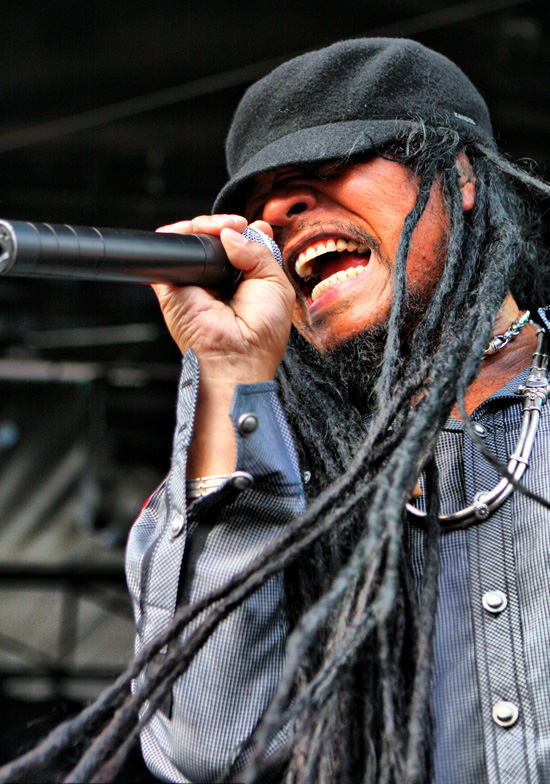The photograph captures a man engrossed in singing with his right hand gripping a black microphone that has a silver head. He sports a black felt cap and has long black dreadlocks that cascade past his waist. His attire includes a blue, denim-like shirt featuring metal clasps for buttons on both the front and sleeves, where two out of three buttons are undone. Around his neck are two thick, double-banded silver necklaces. The background, although blurry, reveals scaffolding and structural supports, indicating he is performing on a stage, likely at an outdoor venue during daytime due to the visible natural light. The image focuses on the man from his upper stomach upwards, though one arm is partially cut off at the edge of the photograph. His facial hair includes both a beard and a mustache.